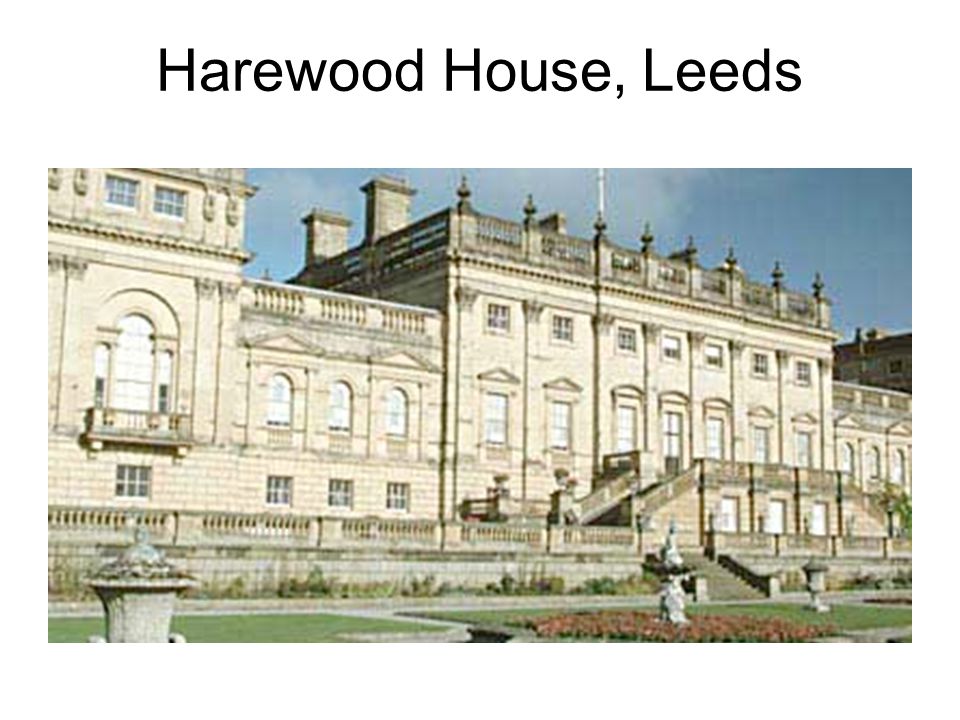This image captures the grandeur of Harewood House in Leeds, England, showcasing its historic and ornate architecture. The building, reminiscent of a pseudo-castle or Victorian mansion, is characterized by its expansive façade made of white and tan-colored stone. The front of the house is punctuated by numerous windows, with a mix of square and arched styles, some of which are sealed off. Above, an intricate railing surrounds a terrace area, potentially once used for guard patrols or leisurely walks, adorned with pointed, decorative features.

In front of the imposing structure, a well-manicured garden stretches out, featuring green lawns, red flowerbeds, and paved walkways. Central to the garden is an ornate design, possibly a statue or fountain, adding to the detailed landscape. Dual staircases lead up to the main entrance, suggesting an impressive approach with about 50 steps. The overall design conveys a sense of historical importance and aesthetic elegance, making Harewood House a notable landmark possibly used for political or public purposes.